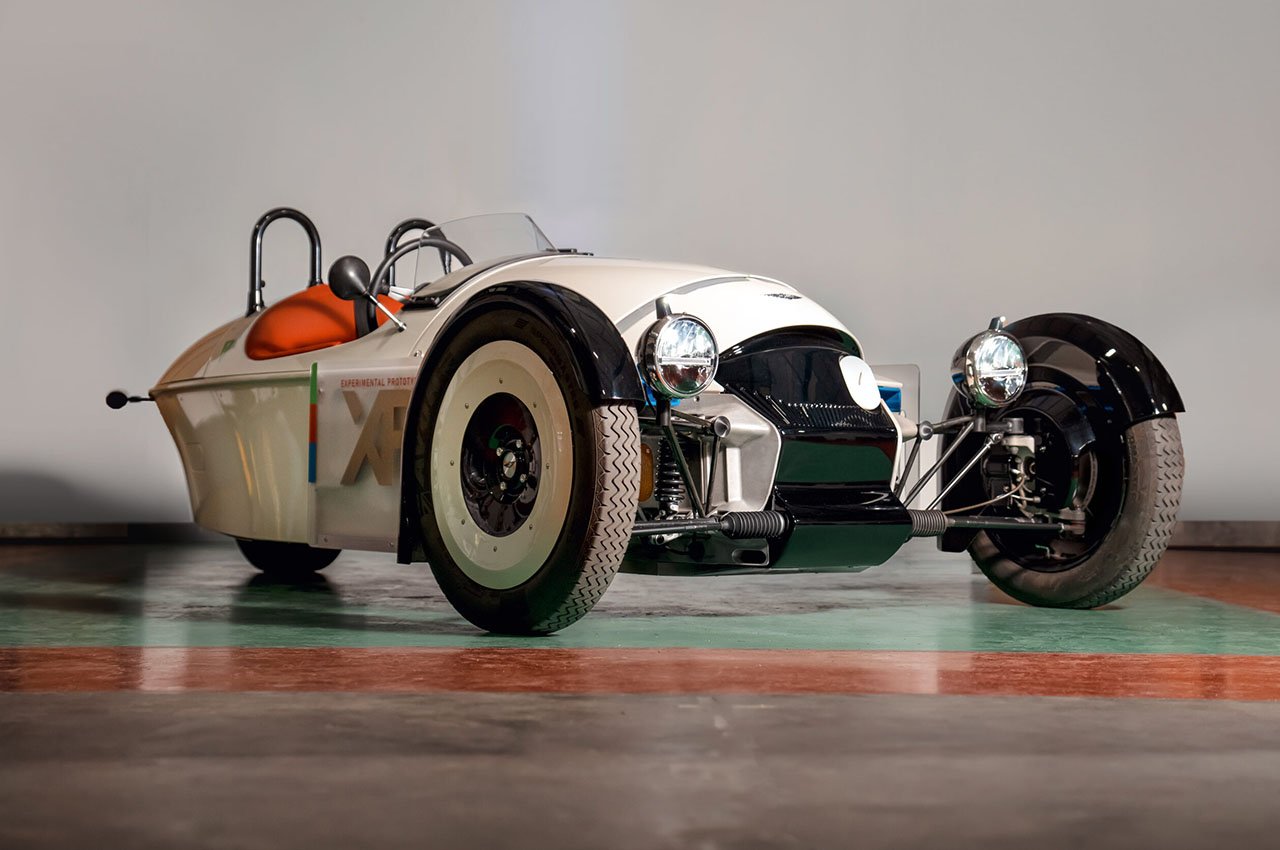This image showcases a detailed model of an old-fashioned, three-wheeled speedster race car on a showroom floor. The vehicle has a sleek, torpedo-like shape with white bodywork and two enormous wheels at the front, nearly as tall as the vehicle itself, adorned with silver hubcaps. The black fenders at the front feature headlights mounted on beams. The single seat is a vivid red or bright orange, with a short, clear windshield in front of it, and a black roll bar behind for safety. The car's minimalist grille and exposed framework between the two front wheels highlight its vintage design. The rear features one wheel at the center, partially visible from beneath the vehicle. Gold lettering, possibly 'XF' or 'XP,' embellishes the side of the car, adding a touch of elegance. The model sits on a uniquely colored tiled surface with shades of blue-green, orange, and lilac, against a white wall background with grayish trim.